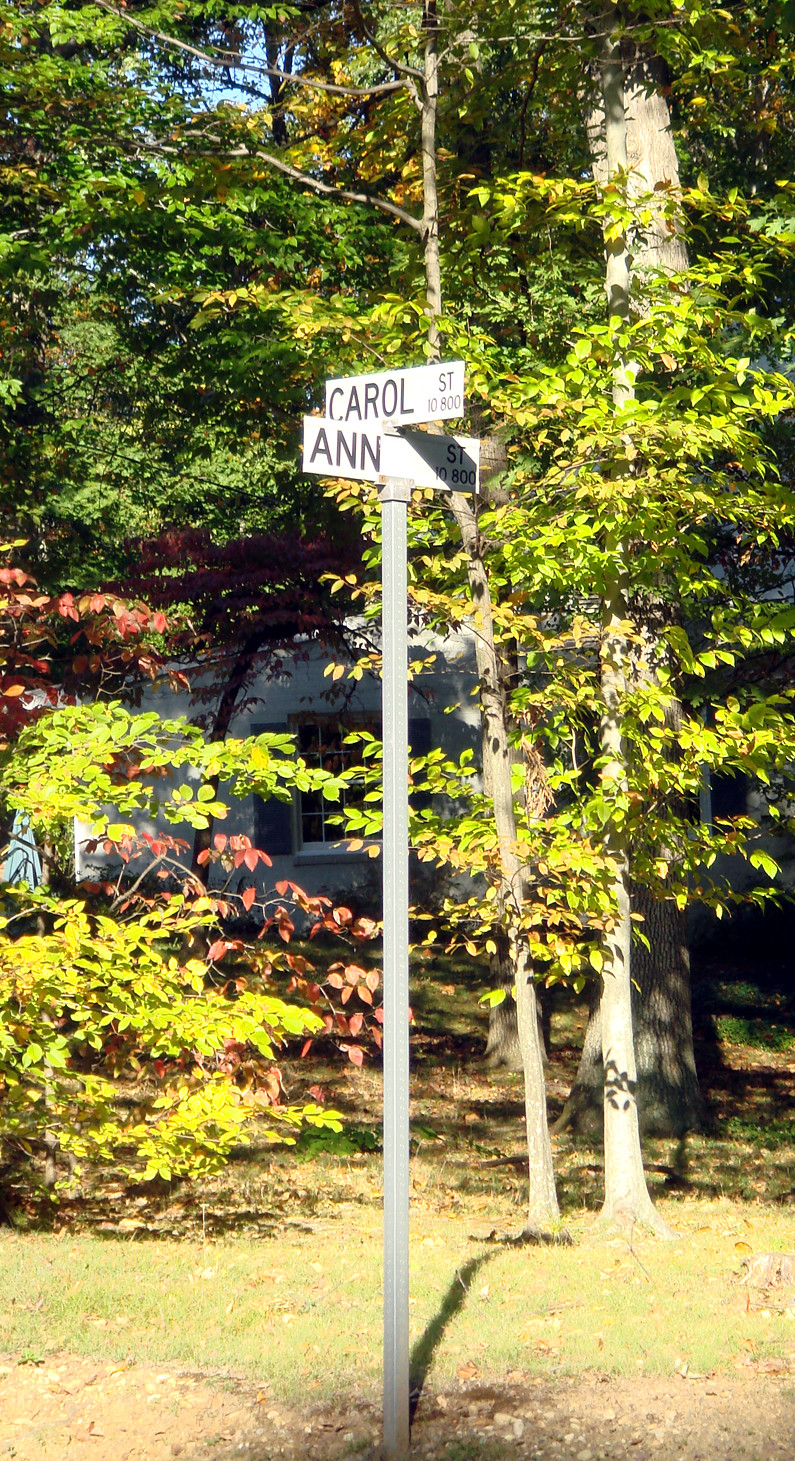This vertical photograph captures a street sign anchored by a silver, square pole against a vibrant, natural backdrop. The setting appears to be outdoors, surrounded by large trees and dense shrubs showcasing a rich tapestry of foliage in shades of green, light green, orange, and red, indicating the beauty of a transitional season. Below the lush canopy, the ground is covered with verdant grass. Atop the metal post, two intersecting white rectangular signs display street names in a clean, legible font. The upper sign reads "Carroll Street 10-800," while the lower sign indicates "Ann Street 10-800," marking the cross streets in this picturesque, foliage-rich scene.